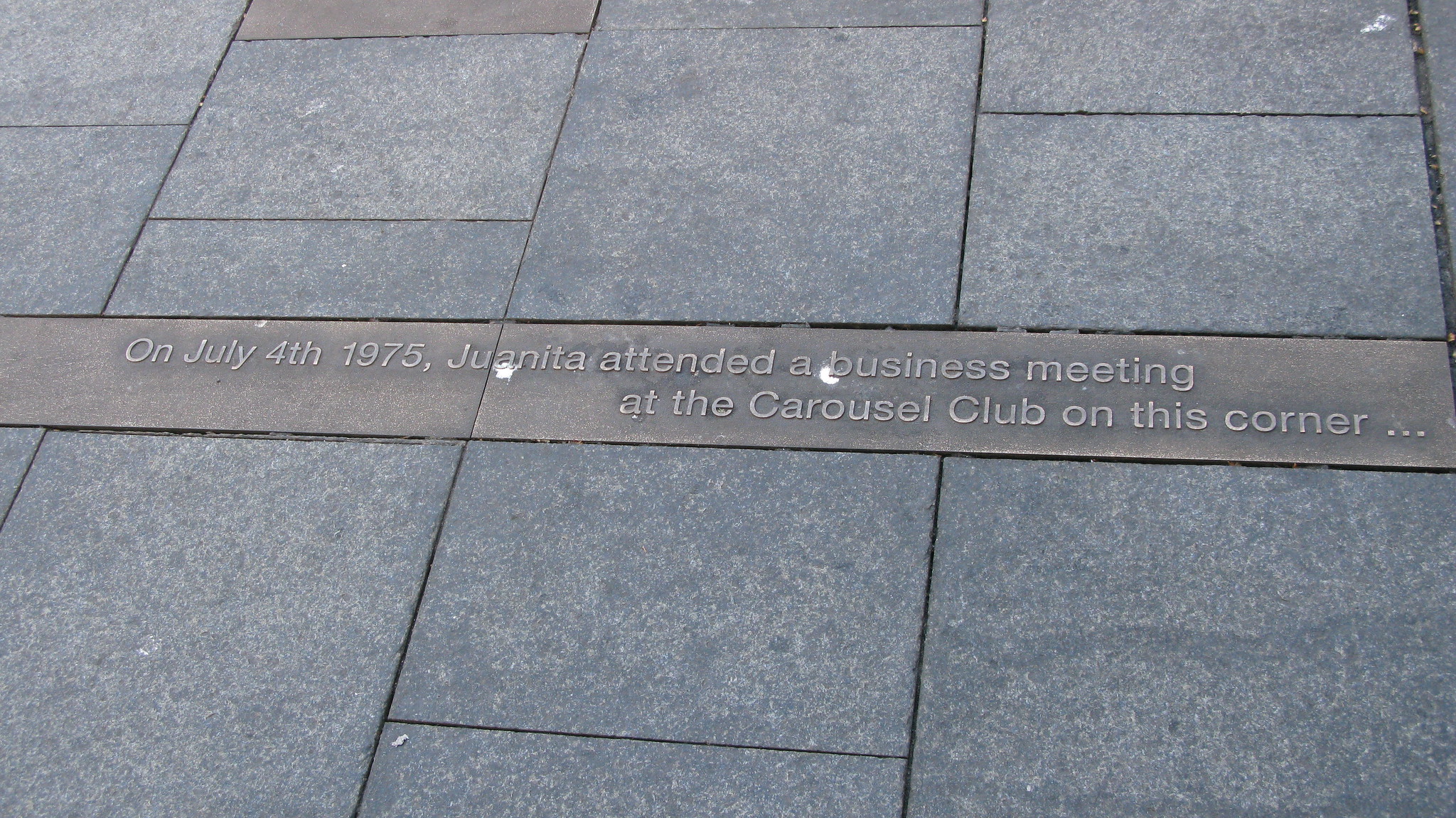The image features an outdoor scene of concrete pavement interlaid with varying tiles in shades of brown and gray, set in a mixed pattern of rectangles and squares. Dominating the center of the image, there is a metal plaque embedded into the pavement. The plaque bears an inscription in light gold lettering that reads, "On July 4, 1975, Juanita attended a business meeting at the Carousel Club on this corner..." The text suggests that this location holds particular historical or personal significance, possibly recognized by local residents. The surrounding pavement reveals a few cracks filled with leaves and debris, adding a touch of natural imperfection to the scene.